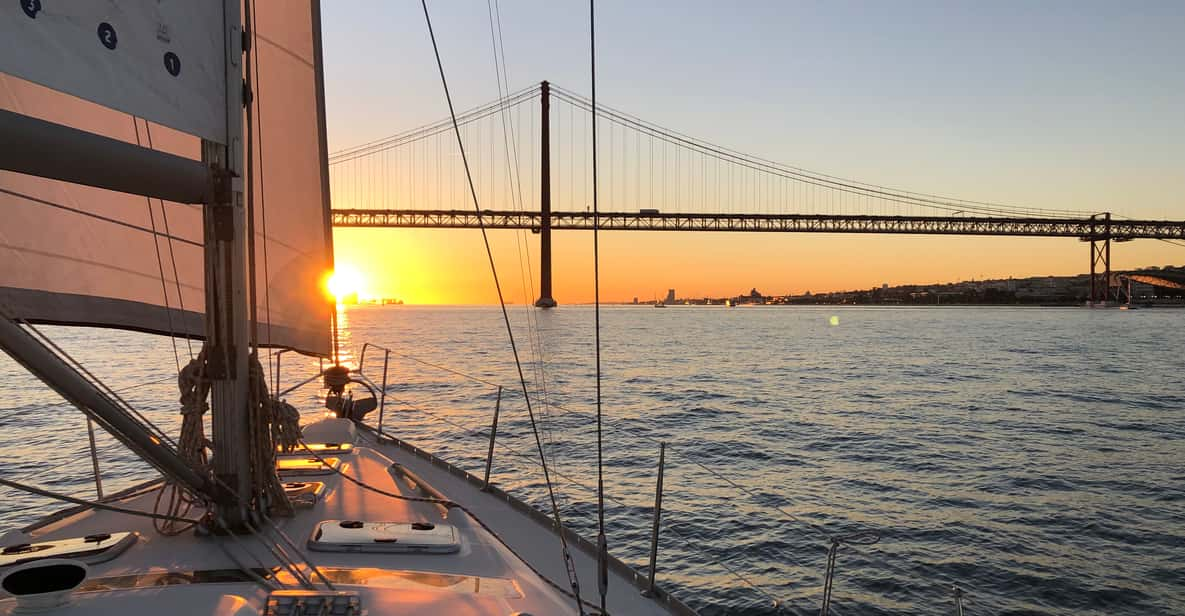In this tranquil portrait-mode photograph, a sailboat navigates on a vast body of water, likely an ocean. The sailboat, largely white with a prominently raised sail marked by dark pink and black stripes, commands the left side of the image. The vessel's mast is visible, though there are no people on board, reinforcing a serene atmosphere.

The centerpiece of the image is a grand suspension bridge, its metal cables sharply defined against the sky. The bridge stretches across the water, with a few cars seen traversing it, and disappears towards a distant, dark mountain on the left. This mountain, almost island-like, emerges from the water and adds to the serene complexity of the scene.

The sunset, positioned slightly left of center at the horizon, bathes the sky in vibrant hues of red, blue, and gray, blending beautifully. The surface of the ocean mirrors these colors in a calm tableau. The sun is low, casting a golden glow over the water and the boat, which sails towards this enchanting mix of colors.

To the right of the bridge, there appears to be a modest cityscape, characterized by some greenery and trees marking its boundary. This, coupled with a few other boats far in the background, completes a strikingly peaceful and detailed scene, capturing the quiet elegance of the sailboat's journey towards the setting sun.